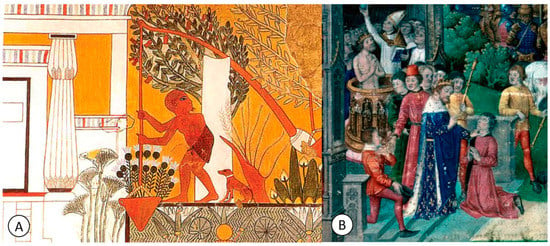The image is divided into two distinct parts, labeled Box A and Box B. 

Box A features an old illustration with an ancient, possibly Egyptian, aesthetic. Central to this part is a reddish-orange child, dressed in a loincloth, who appears to be operating a pulley system to lift some flowers. The boy's face is turned backward, and a small red dog stands beside him. He holds a wooden tool with an orange triangular head, and the scene is set against a building adorned with columns and detailed trim around the doors. Additional elements include a tree or bush and various plants, adding to the historical ambiance.

Box B portrays a more intricate and detailed image resembling a classic painting. This scene showcases a royal figure, likely a king, dressed in a velvet blue cape with a white stole around his neck and a golden crown on his head. The king is in the process of knighting a kneeling individual. Surrounding the main figures are various court attendees, including possible jesters and a person in the background with hands in a prayer position. The setting features stairs, green bushes, and a backdrop with a circular tower-like structure where more people are gathered, some wearing distinctive headpieces.

This combination of illustrations and classical imagery weaves a rich tapestry of historical and cultural symbols, creating a visually captivating scene divided into two distinct yet complementary parts.